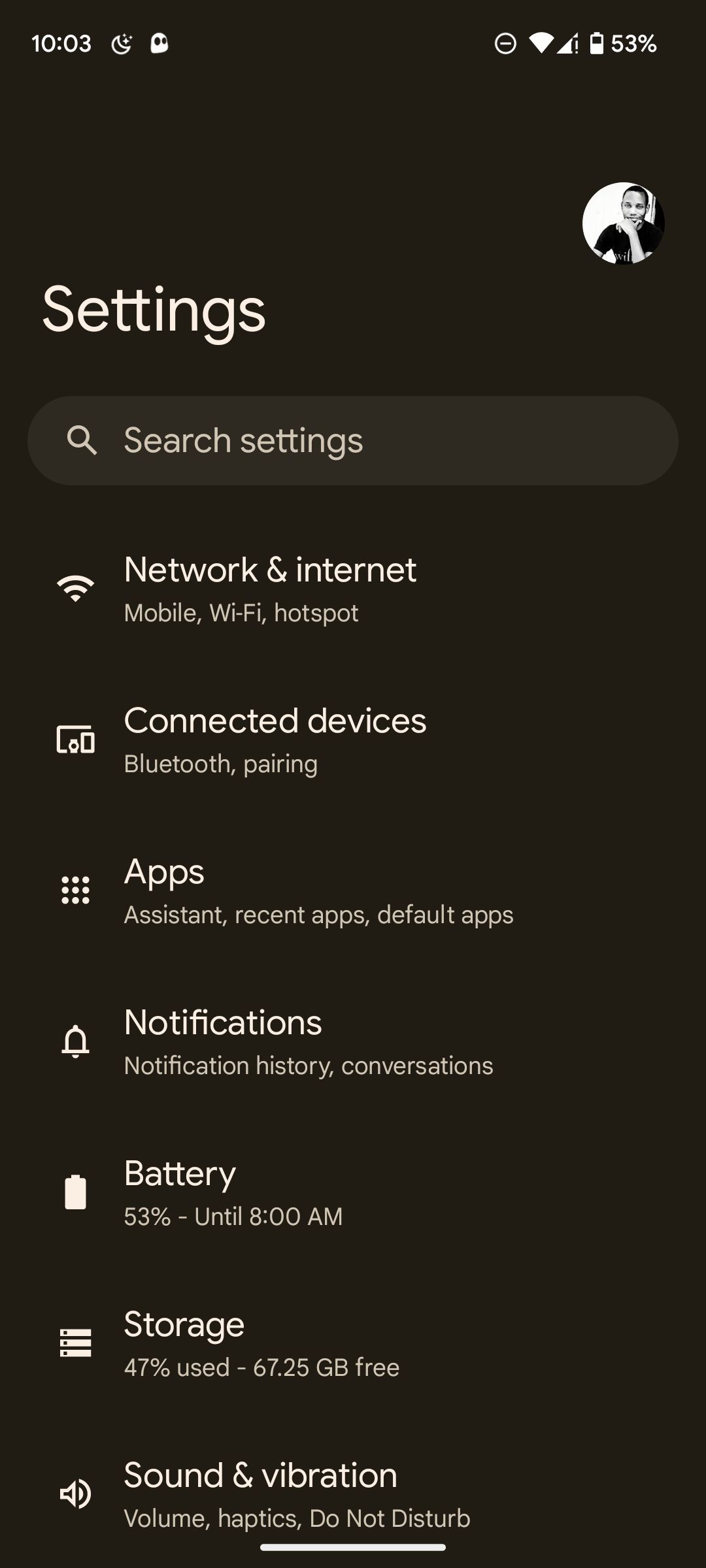This image showcases a smartphone screenshot featuring the device's settings menu displayed against a sleek black background with white text. At the top, the status bar is visible, indicating the current time along with various icons that represent the battery percentage, Wi-Fi signal strength, carrier signal, and other system statuses. Just below the status bar is a user's profile picture alongside the label 'Settings'.

A search bar labeled 'Search settings' appears underneath the profile picture, providing quick access to specific settings. The main body of the screen presents a comprehensive list of menu items, including:

- **Network & Internet**: Manages Wi-Fi, cellular data, and other network connections.
- **Connected devices**: Options for Bluetooth pairing and other related settings.
- **Apps**: Allows access to recent apps, default apps, and the device's assistant.
- **Notifications**: Displays notification history and settings for managing conversations.
- **Battery**: Shows battery status, including remaining life and charging requirements.
- **Storage**: Indicates storage usage, showing that 47% of the storage capacity is currently utilized.
- **Sound & Vibration**: Provides controls for volume settings and Do Not Disturb options.

Each menu item is clickable, allowing the user to configure their device's settings according to their preferences and requirements. The clear and organized layout of this settings menu ensures easy navigation and management of various aspects of the smartphone.